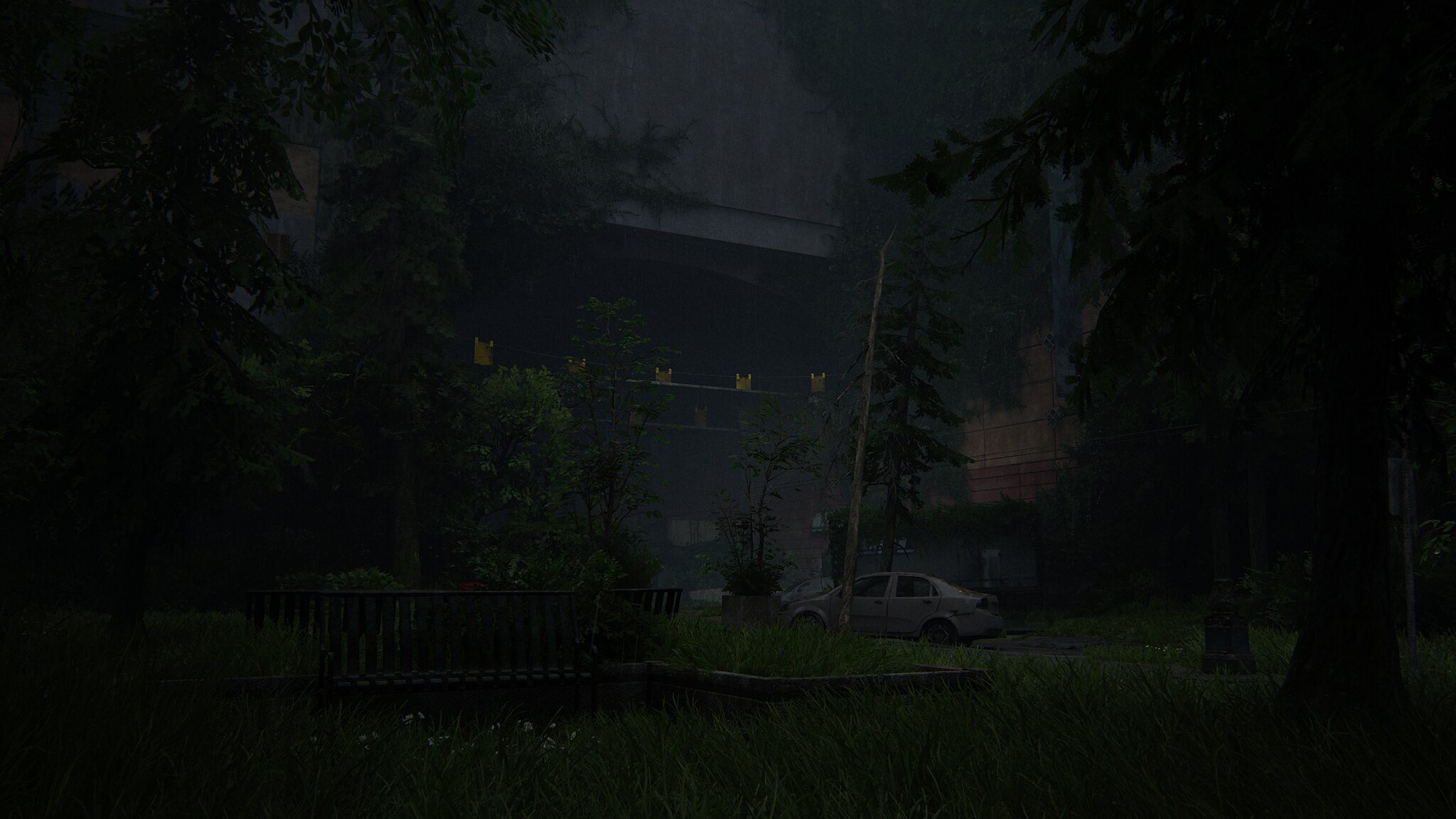This image depicts a screenshot from a video game or possibly a piece of digital or concept art. The scene evokes the post-apocalyptic ambiance reminiscent of games like "The Last of Us" or "Days Gone." The background is shrouded in dark tones, emphasizing the decay and desolation of the world. At the forefront, an abandoned, tan-colored car sits on a grassy road, overtaken by nature as wild grass and forestry reclaim the area. Green trees loom in the background, adding to the overgrown atmosphere. To the side, a bench is visible, with grass sprouting through it, further indicating the long passage of time and neglect that have allowed the environment to flourish unchecked. The overall mood is one of eerie abandonment and nature’s resilience in the face of human absence.